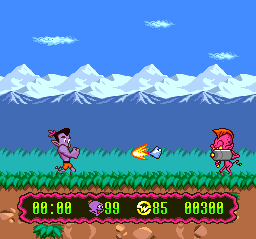In the foreground, a purple character with black hair and orange shorts is seen running toward another character who is red and resembles a devil. The red character is holding a silver box and has launched a fiery weapon toward the purple character, who has his hands up in defense. The scene is set in a mountainous landscape with tall weeds and grass underfoot. Snow-covered white mountains rise in the background beneath a blue sky dotted with puffy clouds. Below the action, an oval scoreboard displays green digits: the purple character has a score of 99, and a yellow image has a score of 85. The backdrop of the scoreboard is a dirt color with scattered rocks.